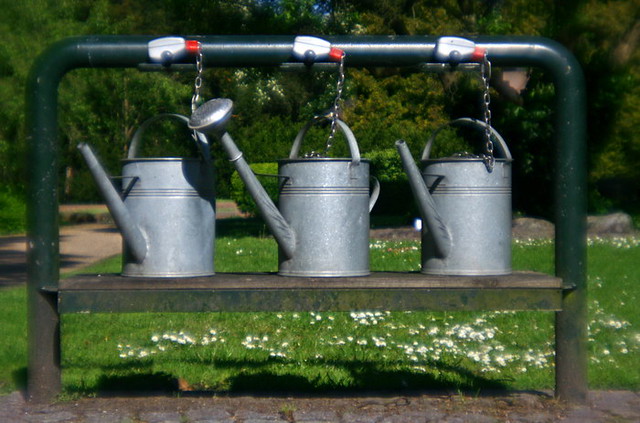This outdoor photograph captures a quaint garden scene showcasing three galvanized metal watering cans, each secured with a chain to a green, inverted U-shaped pipe structure. The watering cans, which feature handles arching over their tops, are displayed on a green metal shelf near the bottom of the U-shaped frame. Two of the cans have open spouts, while the middle one is distinguished by its sprinkler-type spout. Behind the watering cans, the background is lush with vibrant green grass scattered with small white flowers, flanked by a row of trees with varying foliage including green and yellow leaves. Additionally, the scene includes low bushes, gray rocks, and a noticeable dirt pathway to the left, enhancing the serene, well-tended garden ambiance.